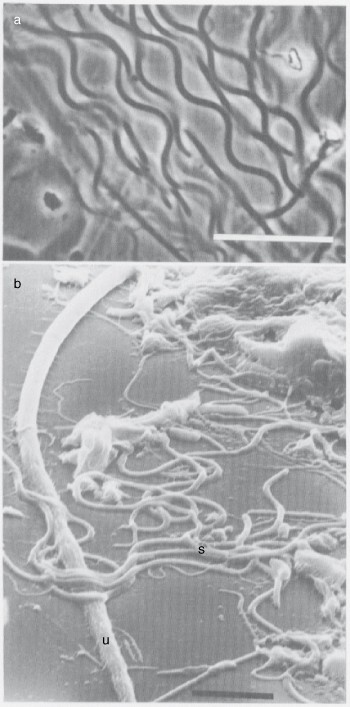The image presents two vertically aligned squares, each showcasing a detailed, zoomed-in view that resembles something observed under a microscope. The top square, labeled with a lowercase white 'A' situated in the top left corner, features a black-and-white photo with various shades of gray. The photo is characterized by intricate, squiggly lines running diagonally from the top left to the bottom right, presenting an extremely close-up perspective that makes further details difficult to discern.

The bottom square, identified by a lowercase black 'B' in the top left, offers a more complex scene. While it retains the extreme close-up nature, it reveals additional elements. There are thicker and white rope-like strands to the left, interwoven with numerous curled strings and scattered splotches, giving the impression of organic material or cellular structures. Adding to the complexity, this square includes lowercase letters: a 'U' positioned towards the bottom right of the center, and an 'S' almost directly in the center but slightly lower. This arrangement of letters insinuates a diagrammatic labeling within the microscopic view. Both squares create a visually compelling, scientific intrigue, depicting intricate textures and structures that invite closer inspection.